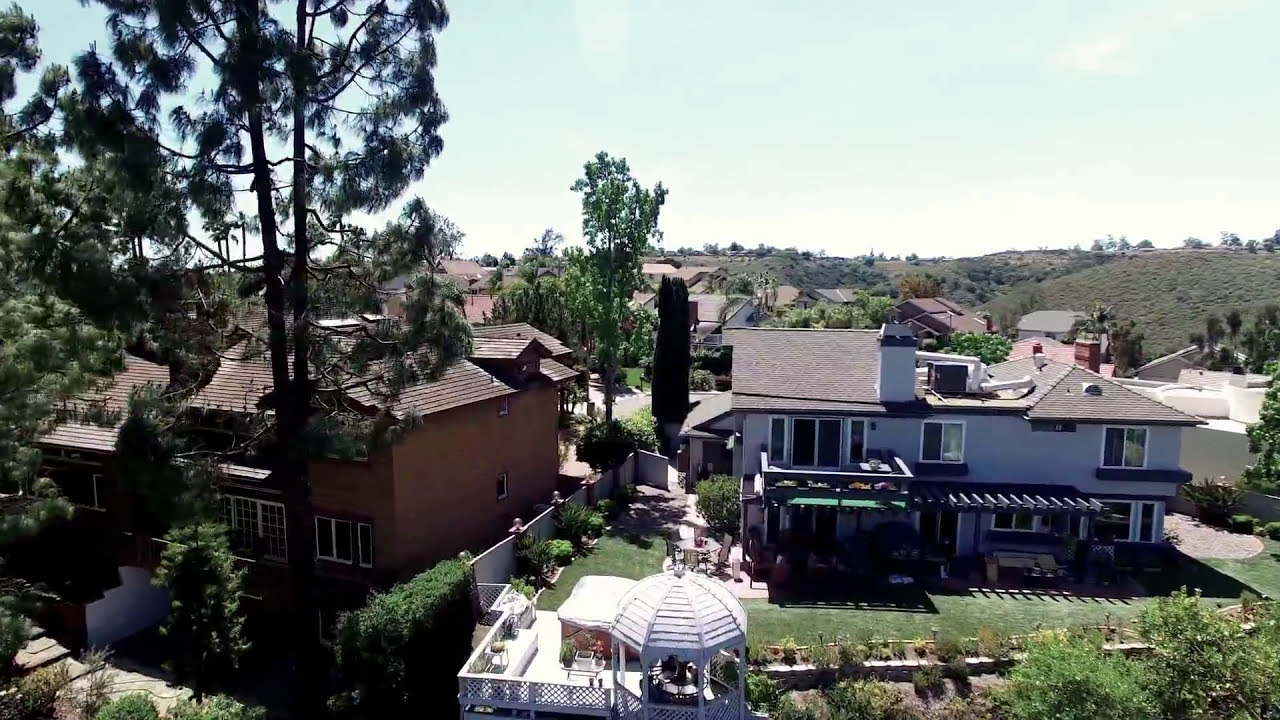This is a detailed aerial view of a suburban neighborhood set against a backdrop of rolling hills and abundant greenery. In the foreground, there's a spacious fenced-in yard featuring a charming gazebo deck outfitted with a hot tub. This property is adjacent to a large house, which appears either light blue or white, the latter being more likely given the angle of sunlight. To the left, there's another sizable house constructed of brick with a dark brown roof, partially obscured by hedges and a fence. This neighboring house has a smaller yard filled with various bushes and smaller trees. Further back, a tree line demarcates the boundary between these homes and the distant roofs of other houses scattered throughout the neighborhood. The sky overhead is clear but punctuated with a few light, white clouds, enhancing the tranquil, daytime ambiance of this residential area.